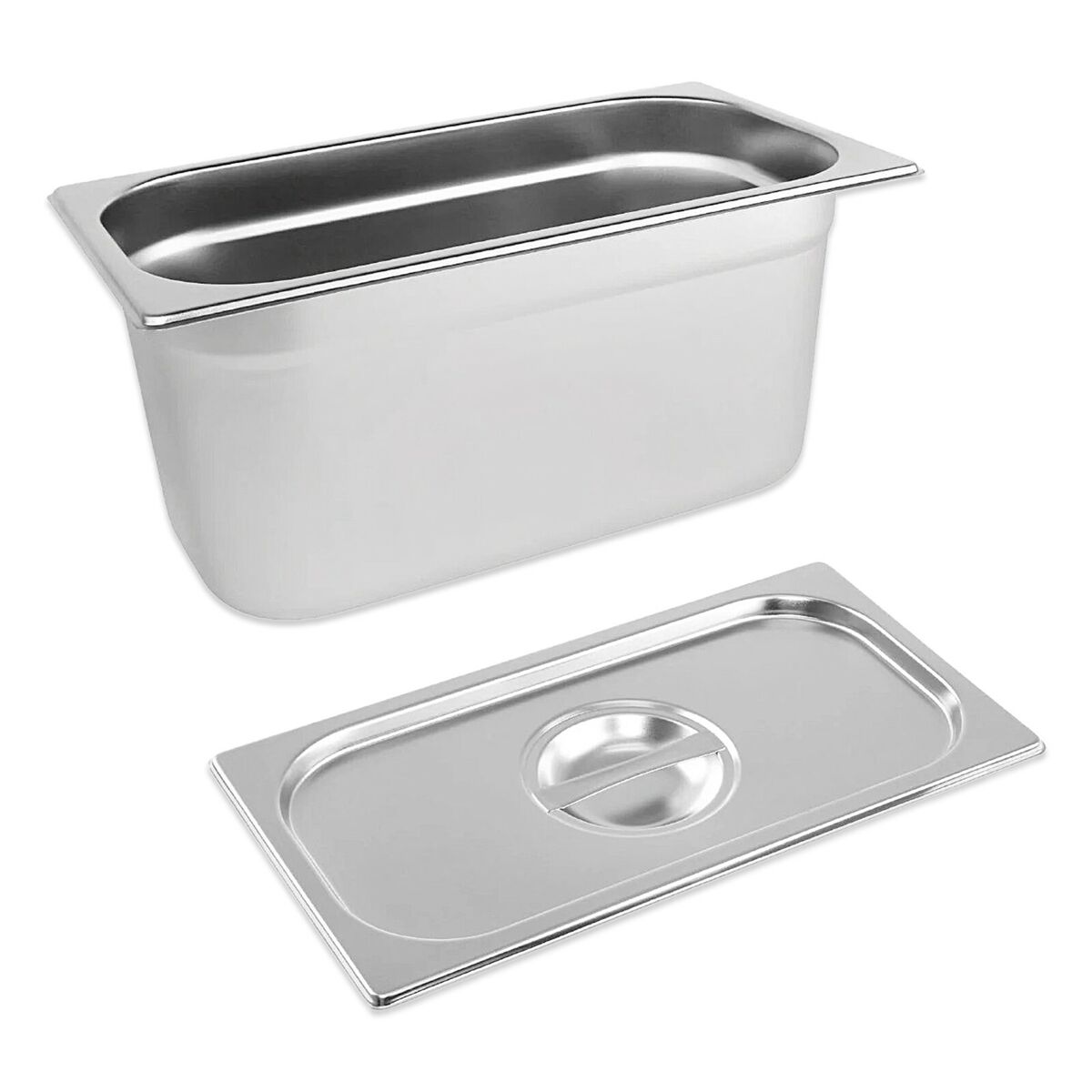This image features a stainless steel steam table pan typically used in professional kitchens, catering, and buffets. The pan is rectangular with rounded sides and bottom edges, designed for easy cleaning. It stands approximately 8 inches deep and 6 inches wide. The interior of the pan is shiny, contrasting with the more matte exterior surface, which won't be visible to the public. Below the pan lies its matching lid, which is flat with a recessed round area in the center, equipped with a bar handle for easy lifting. The lid is designed to fit snugly into the pan, ensuring steam is kept inside to maintain the food's temperature. The entire setup is photographed against a white background from an angle that gently slopes up to the right.